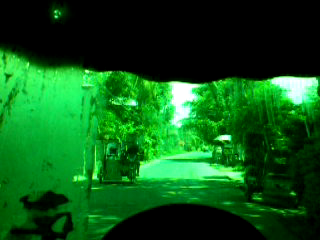This photograph captures a somewhat mysterious outdoor scene with a distinct green hue, suggesting it might have been taken with a green filter. The image seems to be viewed from a concealed position, possibly a hiding spot or under a canopy, as indicated by the black horizontal drape along the top and a semi-circular black shape at the bottom. The setting appears to be a road flanked by trees, with sunlight brightening parts of the road and sky visible in the far background. The photograph shows small vehicles like four-wheelers, construction equipment, and possibly rickshaws or buggies along the sides of the road. A figure, potentially a man with facial hair wearing a beret, is faintly noticeable in the lower left corner. The overall scene evokes a sense of being in a jungle or a less urbanized area, with the green cast adding to its enigmatic ambience.